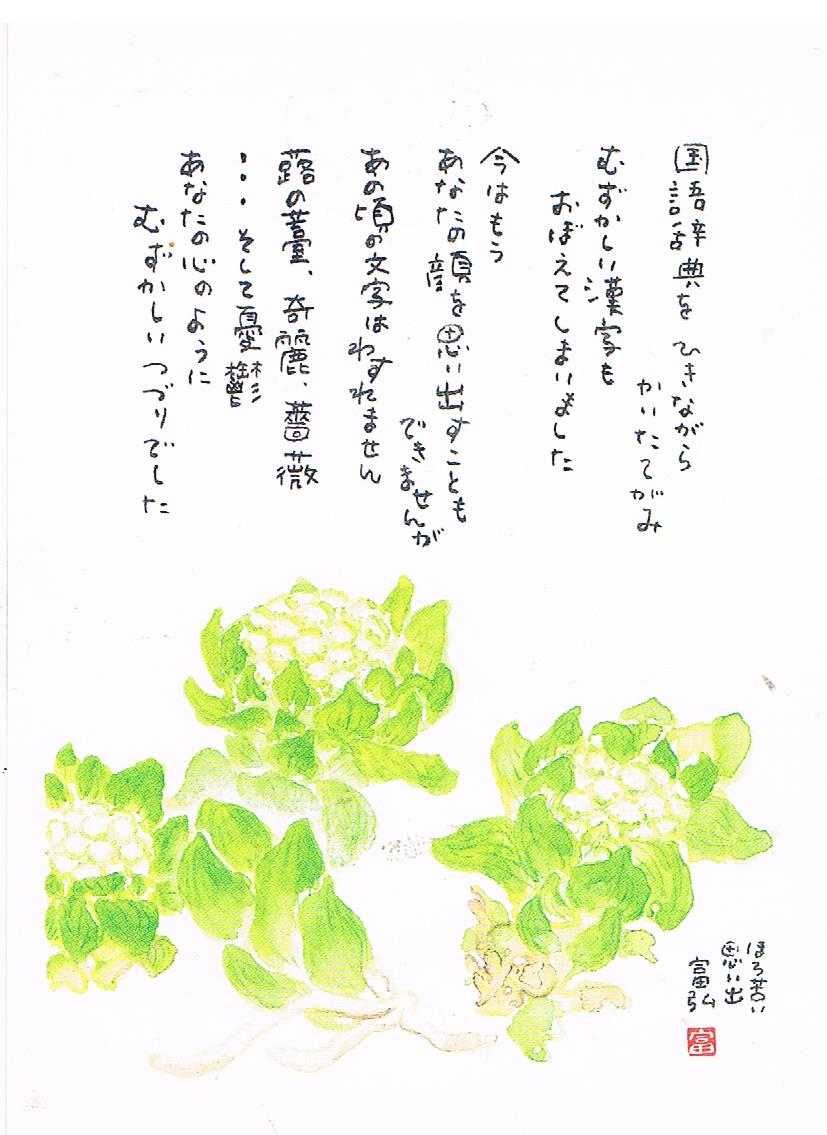This image is a drawing set against a white background. At the top and on the right side of the image, there's handwritten text in black ink, written in an Asian language. The bottom part of the image features a detailed drawing of multiple plants, each with green leaves surrounding white or cream-colored flowers. The central element resembles a cauliflower, with its dense, rounded form, while the green leaves radiate outward, enhancing the resemblance. The scene is intricate, combining botanical elements in a visually appealing manner.